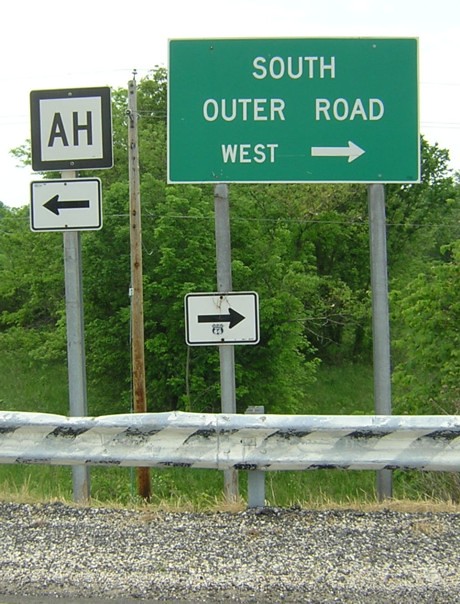In this color photograph of a rural scene, a mix of grassy and gravel areas can be seen flanking the shoulder of a road, which is bordered by a worn, silver guardrail with faded yellow and black diagonal caution stripes. The focal point of the image is a cluster of road signs supported by galvanized metal poles. The primary sign is a large green highway sign with white lettering that reads "South Outer Road West" and features a white arrow pointing to the right. Mounted on the left metal pole beneath this sign is a smaller white sign with a black arrow, also pointing to the right. Additionally, someone has affixed a Route 66 decal to it.

To the left, another galvanized pole supports a square white sign with black borders and the letters "AH" in black. Below this is another white sign with a black arrow pointing to the left. The scene is set against a backdrop of lush green trees, interspersed with patches of brown grass, and a single wooden utility pole with outstretched power lines. The sky is a muted, washed-out light gray, adding a subtle contrast to the vivid greenery of the landscape.